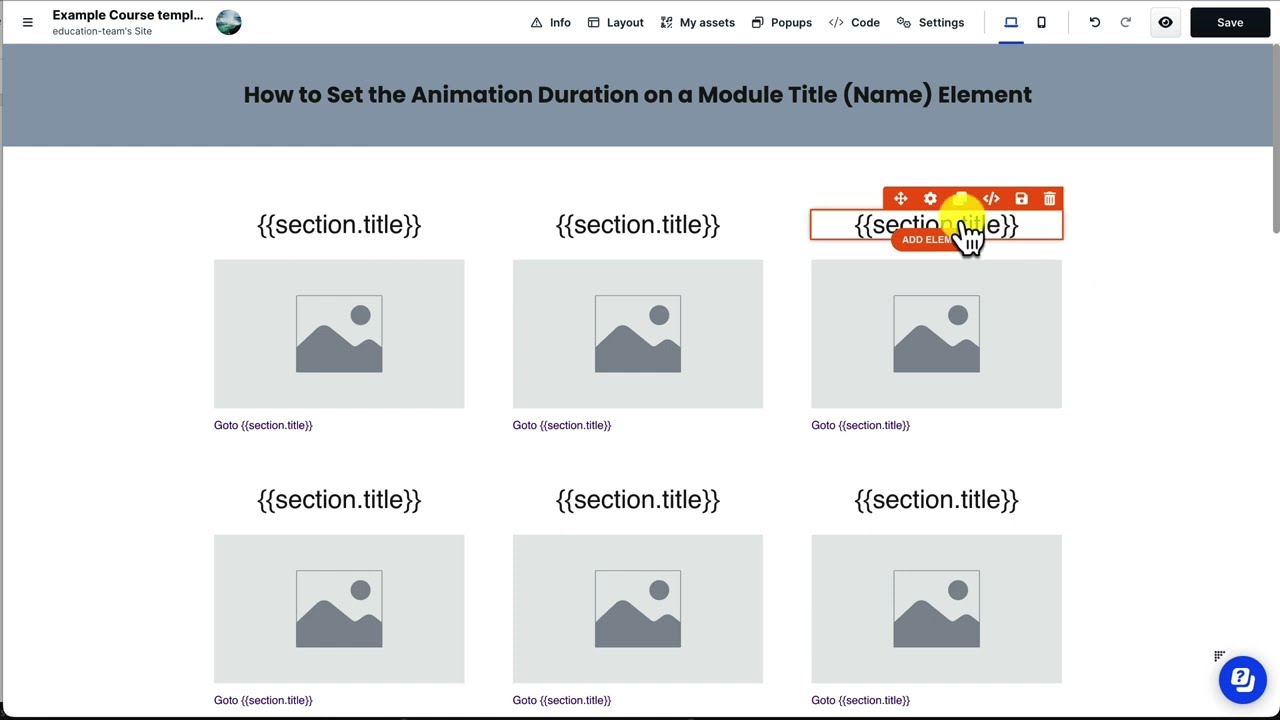The image showcases a slide from an unfinished educational program interface intended for teaching computer skills. Dominating the upper left corner are the words "Example Course Template." Near the top, in a gray bar with black text, is the title "How to Set the Animation Duration on a Module Title, Name Element." The primary section of the screen is white, featuring a 2x3 grid of six placeholders meant for images, each labeled with "Section Title." The top-right placeholder in the first row is highlighted, showing icons for move, settings, and copy actions, alongside a hand cursor indicating selection. Below a placeholder is another "Section Title" label. 

Towards the bottom-right is a blue help icon marked with a question mark. The image predominantly uses gray and white, with additional colors including black, red, yellow, and blue. Top menu options include "Info," "Layout," "My Assets," "Pop-Ups," "Code," and "Settings," with a "Save" button positioned in the upper right. Navigation buttons for forward and backward functions are also present, indicating an interface still under development.